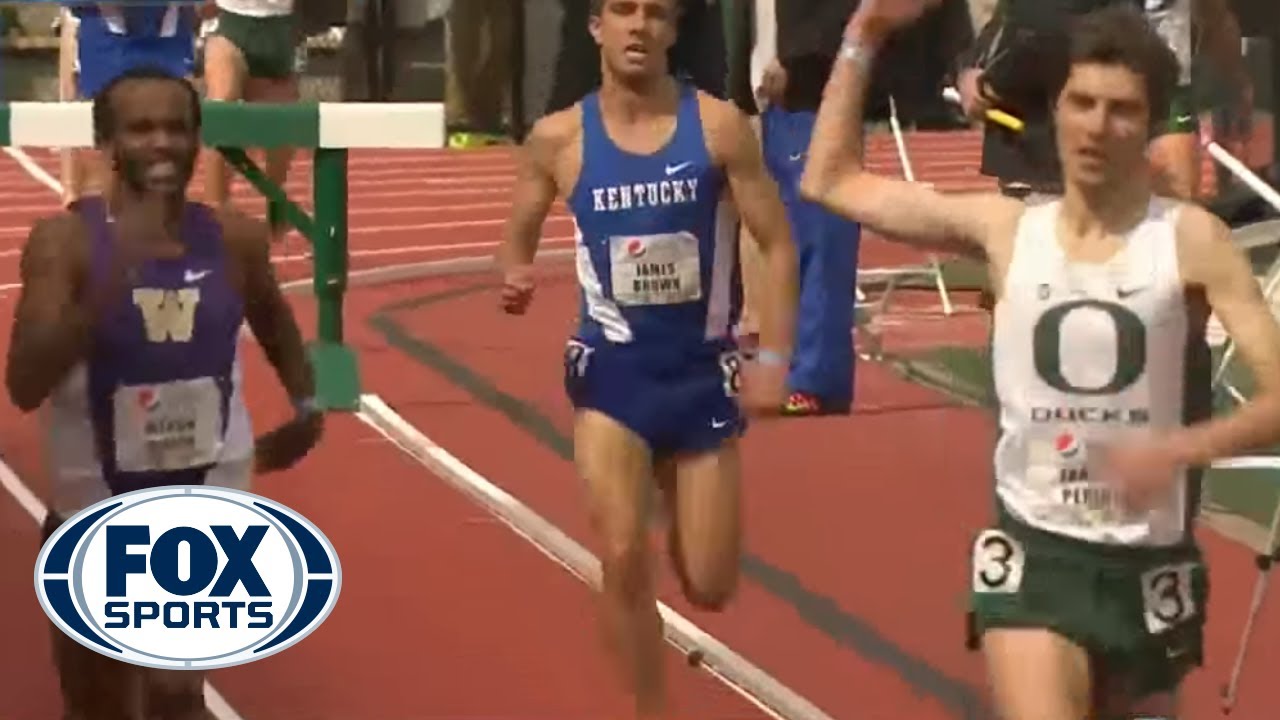This image captures a college track meet featuring three athletes in mid-race, each representing different universities, with the Fox Sports logo in the bottom left corner. The runner on the far left is darker toned, dressed in a purple uniform with a giant gold 'W' on his chest, indicating he is from Washington. The middle athlete, who has a fairly tan complexion, dons a dark blue outfit with the word 'Kentucky' and a Nike logo on his chest. The third runner, on the far right, has fair skin and wears a white and green uniform with a rounded 'O' above the word 'Ducks,' identifying him as an athlete from Oregon. The background reveals a red and white track along with green and white hurdles, and various other athletes and groups of people. The image is quite pixelated and of poor quality, yet clearly depicts the intense competition among the runners.